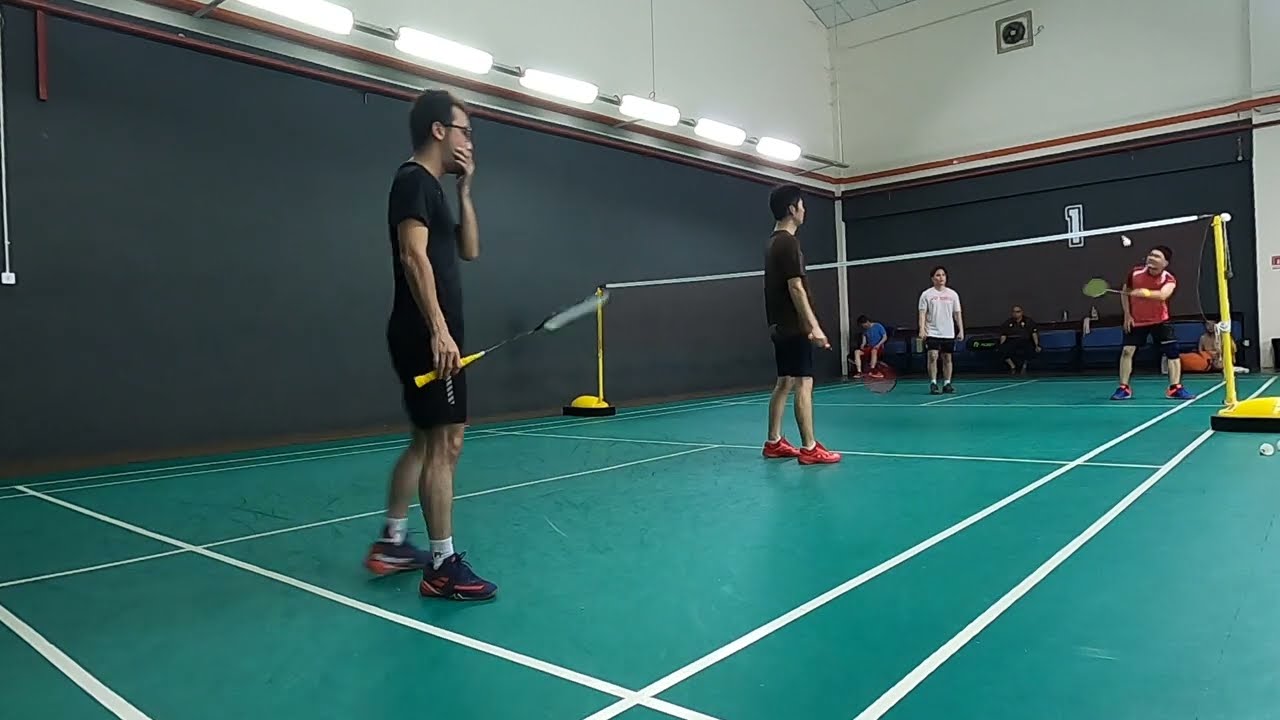The image captures an indoor badminton court with bright green flooring marked by white lines. A white net is held up by yellow poles in the center of the court, dividing the playing area into two sides. The court is encased by dark, possibly black, lower walls, above which lighter-colored walls meet the high ceiling lit by fluorescent lights. In the foreground, two young men wearing black shirts, black shorts, and red-and-black shoes stand on the court's left side. The player closer to us has one hand over his mouth and appears to be looking off-court. Both players grip long rackets with small heads. Across the net, on the right side, two other players are visible: one in a red shirt and black shorts preparing to hit the shuttlecock, and the other in a white shirt standing by, observing. Behind them, near a large number "1" on the wall, a few people are seated, watching the ongoing doubles match attentively. The setting reflects the dynamic atmosphere of a live badminton game.